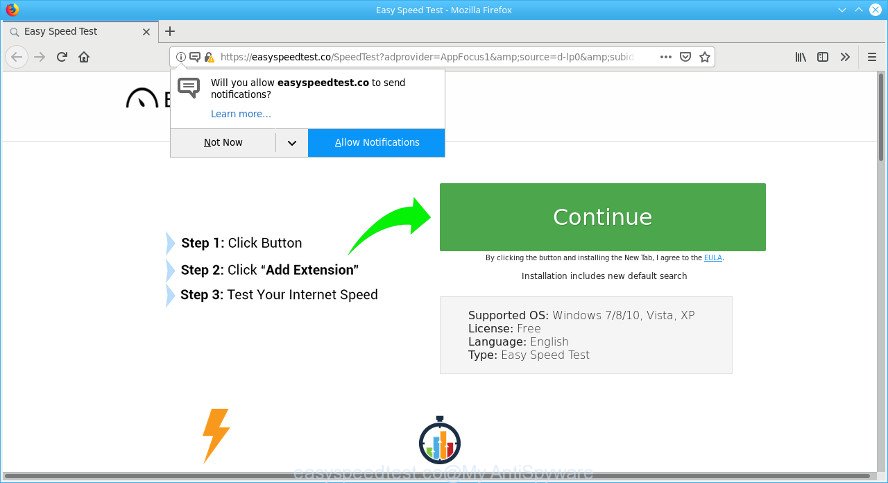This screenshot displays a Firefox browser window open to a website with the URL "https://easyspeedtest.co/speedtest?adprovider=appfocus1&source=d-ipos". The Firefox address bar features an information icon on the far left, indicating the site's security status. Someone has clicked this icon, which has triggered a pop-up dialogue asking, "Will you allow easyspeedtest.co to send notifications?". Below this query, there are two response options: "Not Now" and "Allow Notifications".

The main content of the webpage is visible beneath this pop-up. The page features a step-by-step process to conduct an internet speed test. Instructions on the page read: 
1. Click the button
2. Add the extension
3. Test your internet speed

There is a prominent green arrow pointing towards a "Continue" button, guiding users to proceed with the speed test process. The layout clearly highlights each step and the necessary actions required to complete the speed test.